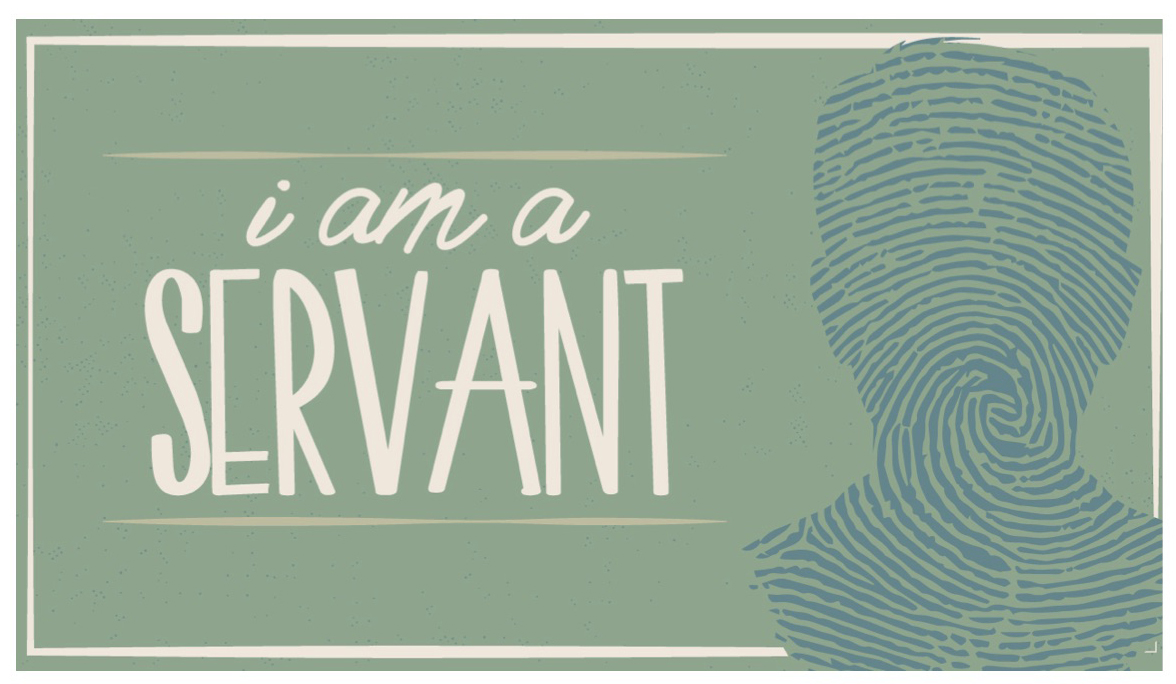The image is likely a sticker design with a layered aesthetic featuring a pale green background bordered by a white outer edge and an inset cream-colored line. Dominating the right side of the image is the silhouette of a man's head, filled with a detailed fingerprint whorl in a blue or dark gray hue. To the left of the silhouette, a motivational slogan reads "I am a servant." The words "I am a" are inscribed in a delicate cursive white font, while "servant" is presented in a larger, thin sans-serif font. These words are framed by thin tan horizontal lines, one above and one below, enhancing the structured look of the design.